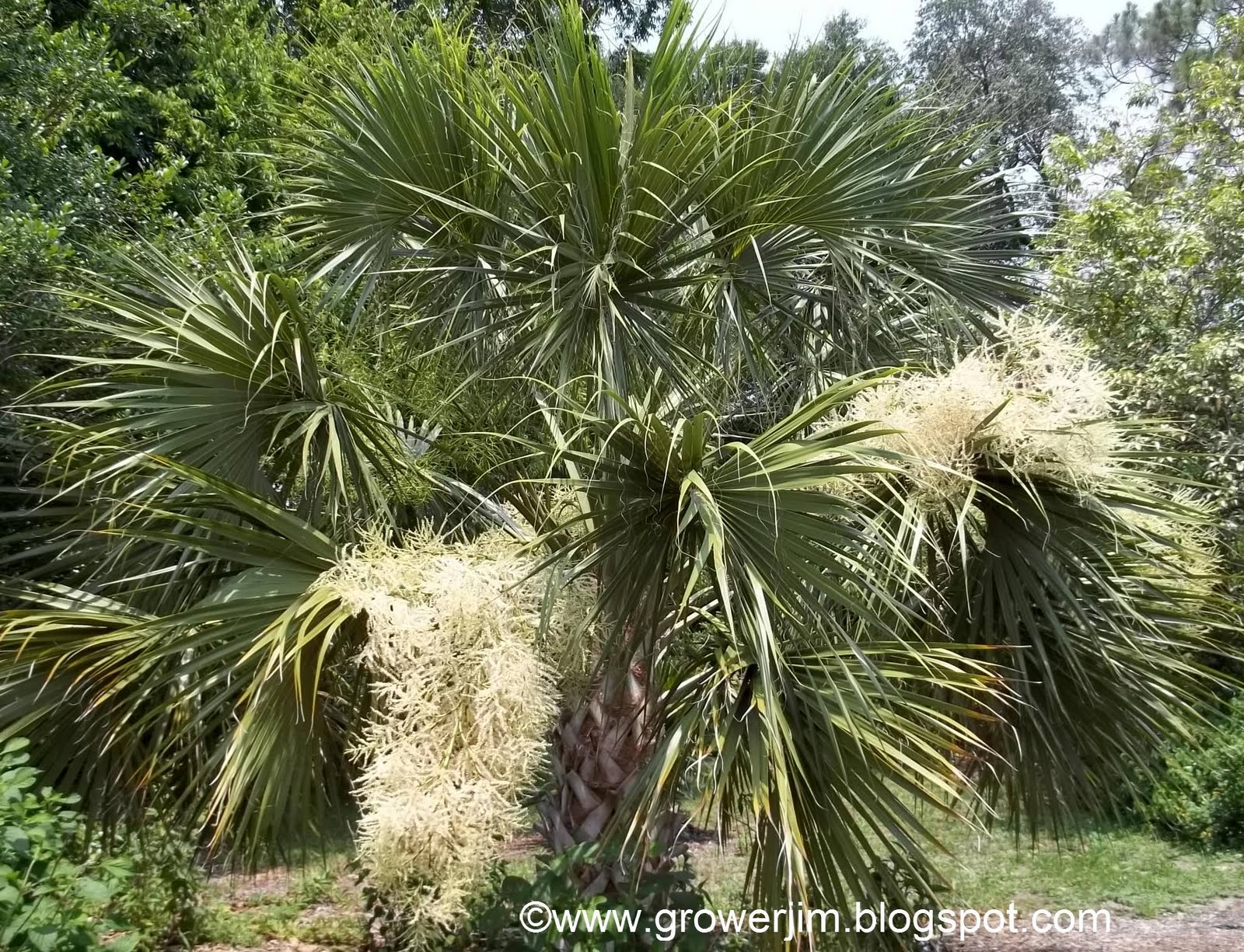This high-quality outdoor photograph, likely taken in a tropical climate, captures the lush and vibrant scene of a garden or backyard. The focal point is a short, large palm tree or plant, characterized by its abundant, fan-like, thin, and pointy green leaves clustered together. The palm also features accents of white Spanish moss draped gracefully on either side. You can spot clusters of yellow flowers adorning the leaves, adding to the rich texture of the scene. The base of the tree is encased in tan, husk-like elements, surrounded by green grass. The background reveals various standard trees with typical leaves, hinting at a diverse ecosystem. The sky peeks through in the upper right with a vivid blue hue, while the ground is sprinkled with assorted vegetation. At the bottom center, the photograph is marked with a copyright symbol followed by the white sans-serif text "www.growergym.blogspot.com," indicating it's sourced from a blog likely centered on gardening or plant cultivation.